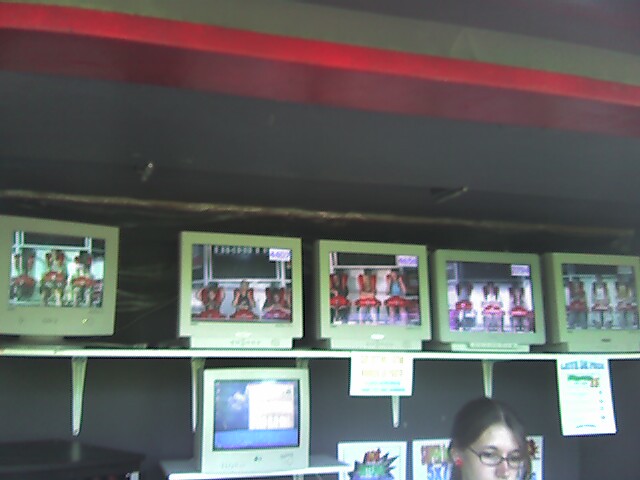This vintage-style photograph captures a nostalgic amusement park booth featuring old box-style computer monitors displaying images of theme park riders. The black back wall sets a stark contrast for the vibrant scene. A green shelf, supported by five green brackets, runs horizontally about a third of the way up from the right, holding five square, older-looking gray computer monitors, each displaying photos of individuals strapped into amusement park ride seats with red straps. The shelving above the monitors includes a small black ledge with a red end, and a touch of green is visible at the very top of the image. Below this setup, an antiquated gray computer monitor, housed on a white shelf, sits next to a black desk's corner edge that partially enters the frame from the left. Three out-of-focus posters hang lower and reveal only their tops. In the lower right foreground, the upper part of a young woman’s face, featuring brown hair and glasses, is visible—potentially a theme park worker. The image exudes a slightly overexposed, vintage charm, reminiscent of old developed photographs.